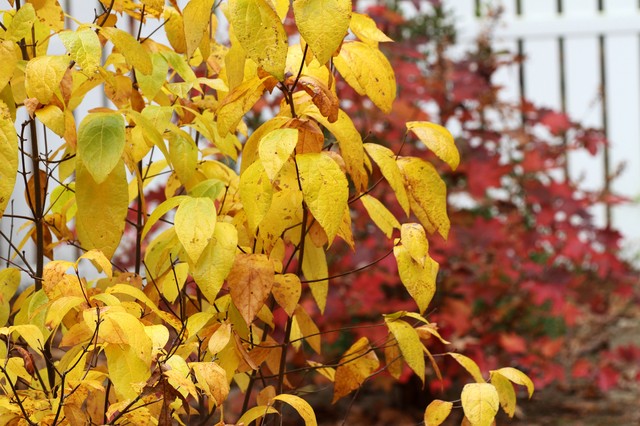The image appears to be taken in a backyard featuring fall foliage. Dominating the left half of the image is a plant with narrow, dark brown stalks and an abundance of golden-yellow pear-shaped leaves, some still tinged with green. A few leaves have deepened into a darker, more orange hue. In sharp contrast, behind this plant on the right side, is another bush of similar shape, but with leaves that have turned a striking blood-red, and a smattering of darker orange. This red-leafed bush is noticeably out of focus, adding depth to the image. In the background, a white painted wooden picket fence, extending horizontally from the left side and continuing across the back, provides a quaint finish to this autumnal scene.